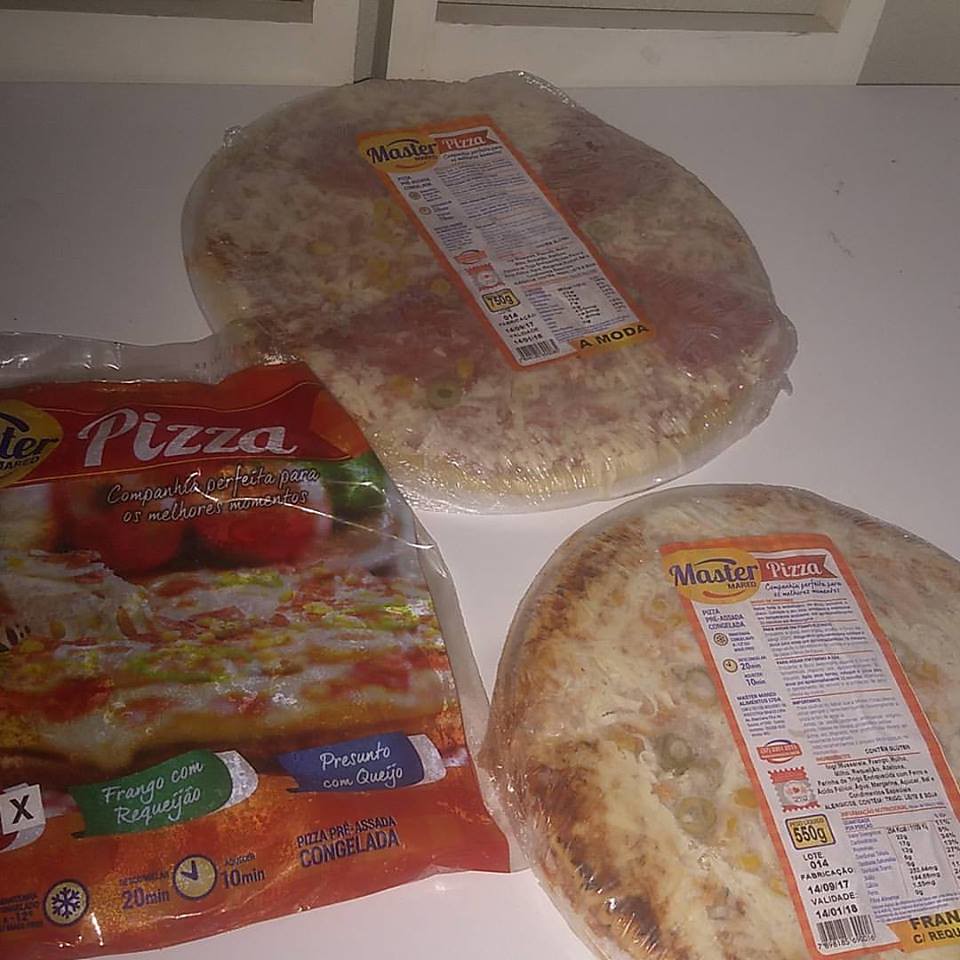This color photograph depicts a white countertop with a smooth, slightly glossy surface, possibly accentuated by flash lighting, which brightens the bottom left corner of the image. Resting on this countertop are three frozen pizzas, each distinctly packaged. The two pizzas on the right are almost identical, encased in clear plastic cellophane, revealing their toppings of cheese, meat, and possibly green peppers or olives underneath. Each of these pizzas bears a prominent label with a white background and orange trim, featuring the brand name "Master Pizza" in purple and white lettering. The label also includes a yellow circle and a red ribbon graphic, as well as nutritional information. 

On the left side of the image is a differently packaged pizza, enclosed in a plastic bag, obscuring the actual pizza itself. This bag showcases a printed image of the pizza and features a red banner at the top reading "Pizza" in white text. Additional text below, suggesting Portuguese, includes phrases like "frango.com," "requeijão," "presunto.com," and "queijo," along with a clock icon indicating a 20-minute bake time. The background of the image fades into a possibly light gray wall and an out-of-frame white window frame at the top. Overall, the details highlight the contrasting packaging styles and labeling of the featured frozen pizzas.